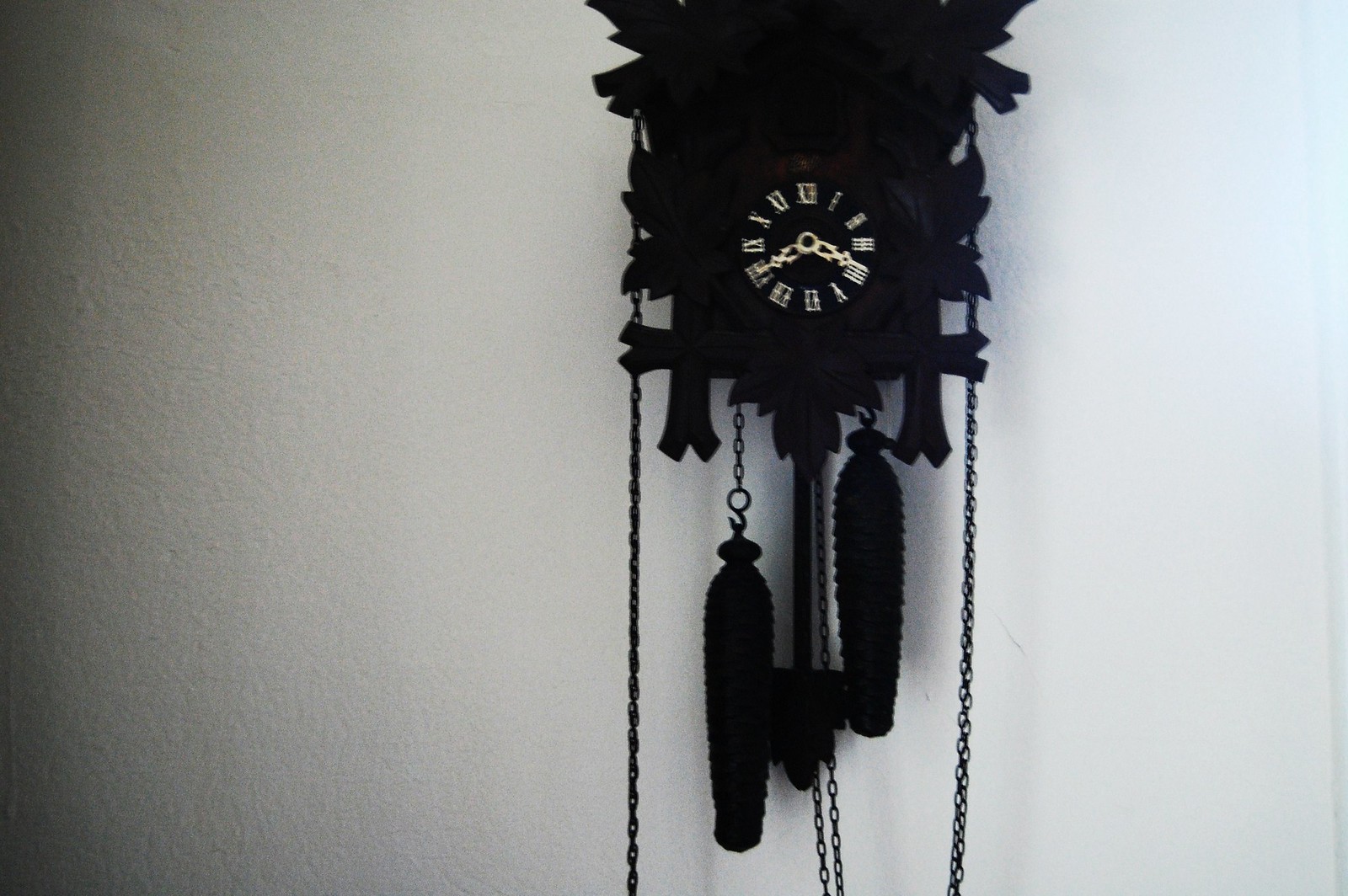The image showcases a light gray, textured wall, typical of a home's interior. Prominently displayed on the wall is an ornate German-style clock, crafted from intricately carved wood. The clock features two chains hanging down, each adorned with elongated pine cone-shaped weights. A pendulum swings at the bottom of the clock. The clock's face is distinguished by white Roman numerals set against a black background, adding a stark contrast to its dark, polished exterior. Although the image is dark, it seems unclear if the clock has a cuckoo mechanism at the top. The time displayed on the clock is 8:20.